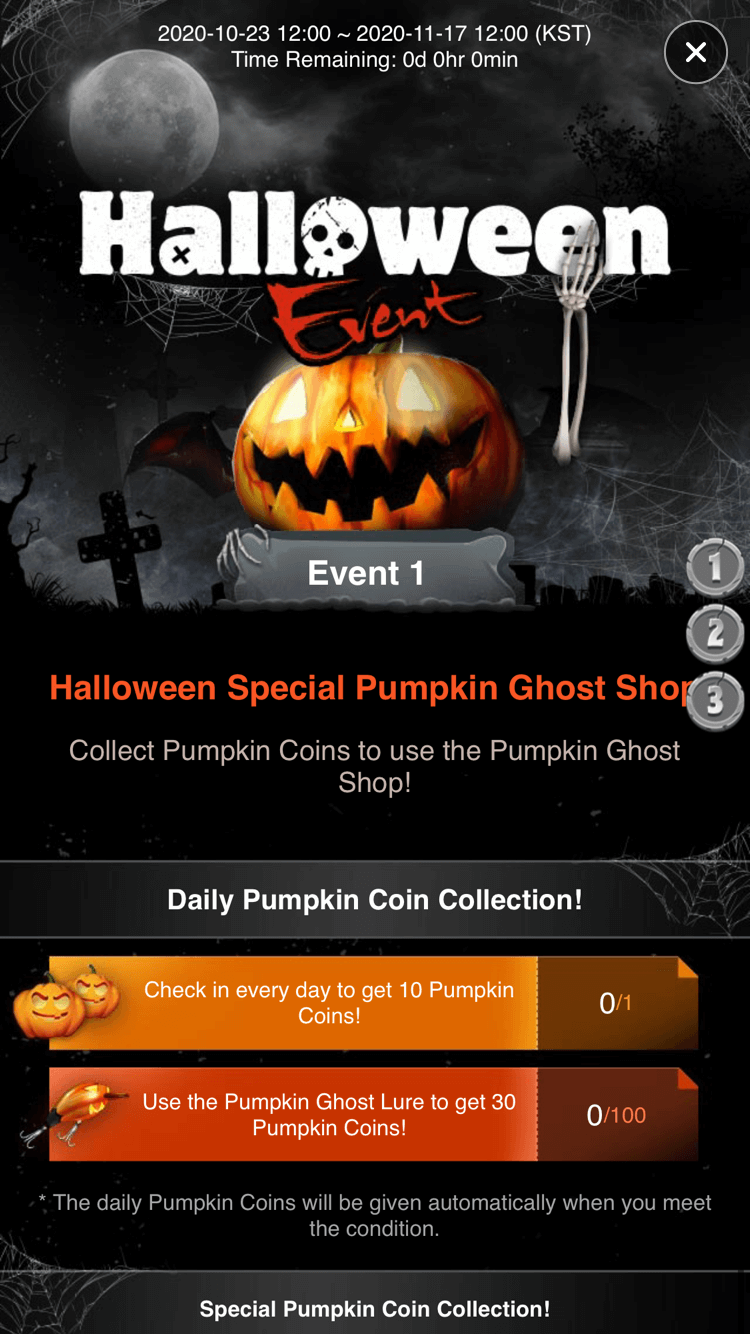The poster displays a haunting graveyard scene, featuring a weathered tombstone under a moonlit, cloudy gray sky. Spider webs lace through the background, complementing the presence of a gnarly, eerie tree trunk. The sky is ominous, lending an air of creepiness to the overall setting.

Prominently displayed, the text reads:

"2020-10-23 1200-2020-11-17 1200 KST. Time remaining: 0 days, 0 hours, and 0 minutes."

The word "Halloween" is written in large, white letters with the 'O' stylized as a menacing skull. Beneath, in bold red letters, it announces an "Event". Nearby, a jack-o-lantern grins wickedly with glowing yellow eyes. Below, a gray box labeled "Event Number 1" describes the event in red letters: "Halloween Special Pumpkin Ghost Shop". Further down, additional text in gray reads, "Collect pumpkin corn to use at the Pumpkin Ghost Shop".

The poster concludes with a segment labeled "Daily Pumpkin Corn Collection," set against an orange box decorated with jack-o-lanterns on the left side, emphasizing the engagement of collecting items daily.

Overall, the detailed and spooky design perfectly sets the mood for an immersive Halloween event.